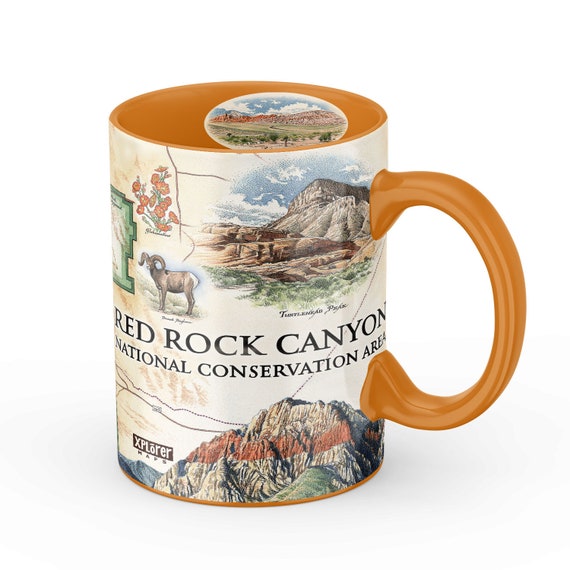The photo features a round coffee mug with a flat bottom set against a white background. The mug has an ochre or mustard yellow interior and handle. The exterior is adorned with detailed artwork related to the Red Rock Canyon National Conservation Area. Centered on the mug in bold black letters is the phrase "Red Rock Canyon National Conservation Area." Surrounding this text are several inset illustrations: a mountaintop showcasing distinct geological layers in varying shades of tan, brown, and reddish clay; a depiction of "Turtleneck Peaks" in smaller letters; a bighorn sheep with large curvy horns; a type of native red flower; and a visual representation of the conservation area's map outline. The mug’s artwork captures the natural beauty of the region with detailed drawings of its iconic formations and native flora and fauna, making it a visually striking piece.